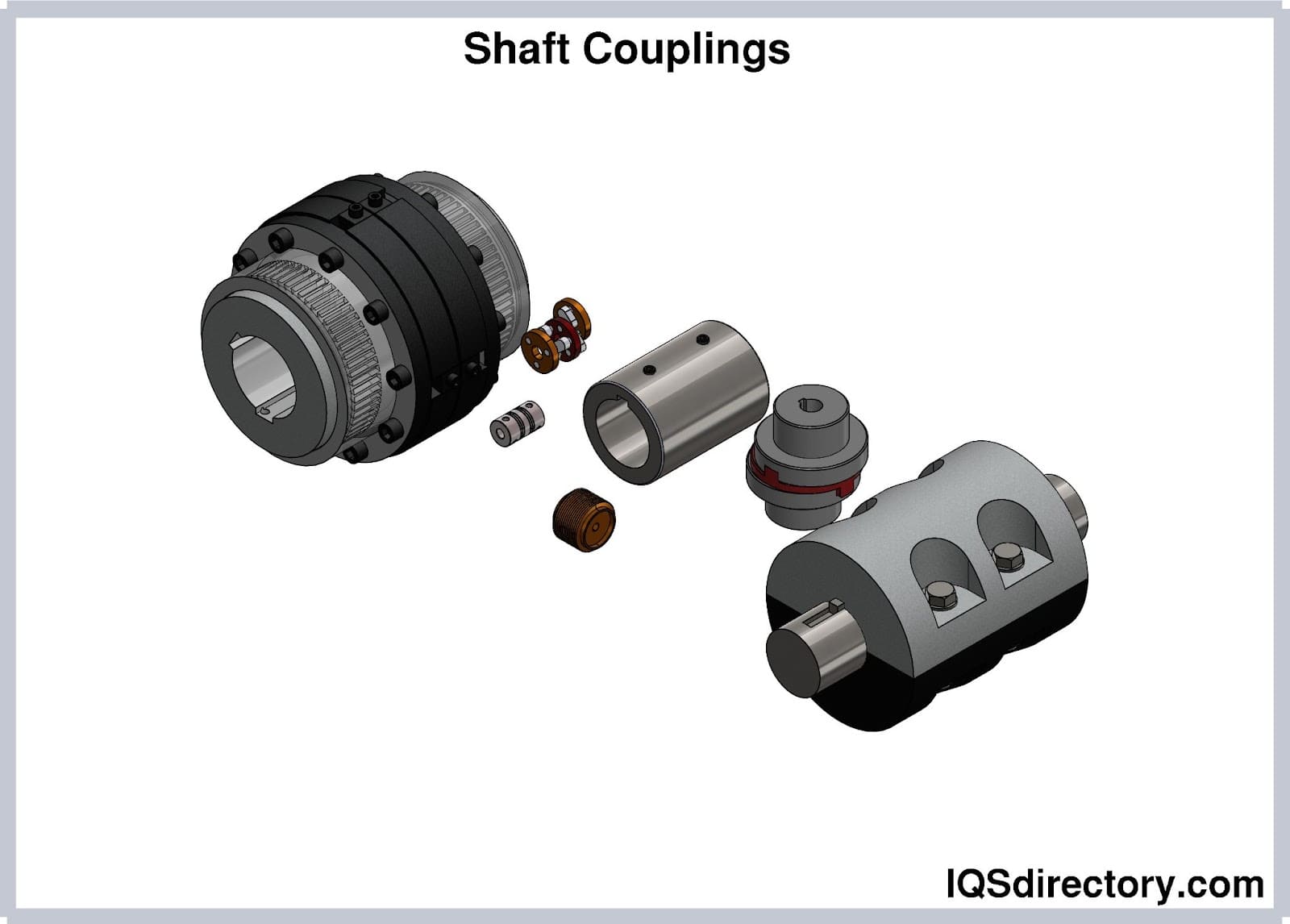The image is a detailed diagram of shaft couplings, arranged diagonally from the top left corner to the bottom right corner on a white background. It features various cylindrical components predominantly in shades of gray and black, with some pieces exhibiting brown and maroon accents. The largest cylindrical piece, located in the top left, includes several cylindrical knobs. Adjacent to it are two smaller components, followed by a cylindrical piece with two holes at the top and a brown cylindrical knob beside it. Further along, a smaller version of the initial cylindrical piece is displayed, and another cylindrical component appears at the end. The image is bordered by a thin gray rectangular border. Text at the top reads "Shaft Components" in black ink, likely in Arial font, and "iqsdirecttrain.com" is noted at the bottom right corner, also in black Arial font.